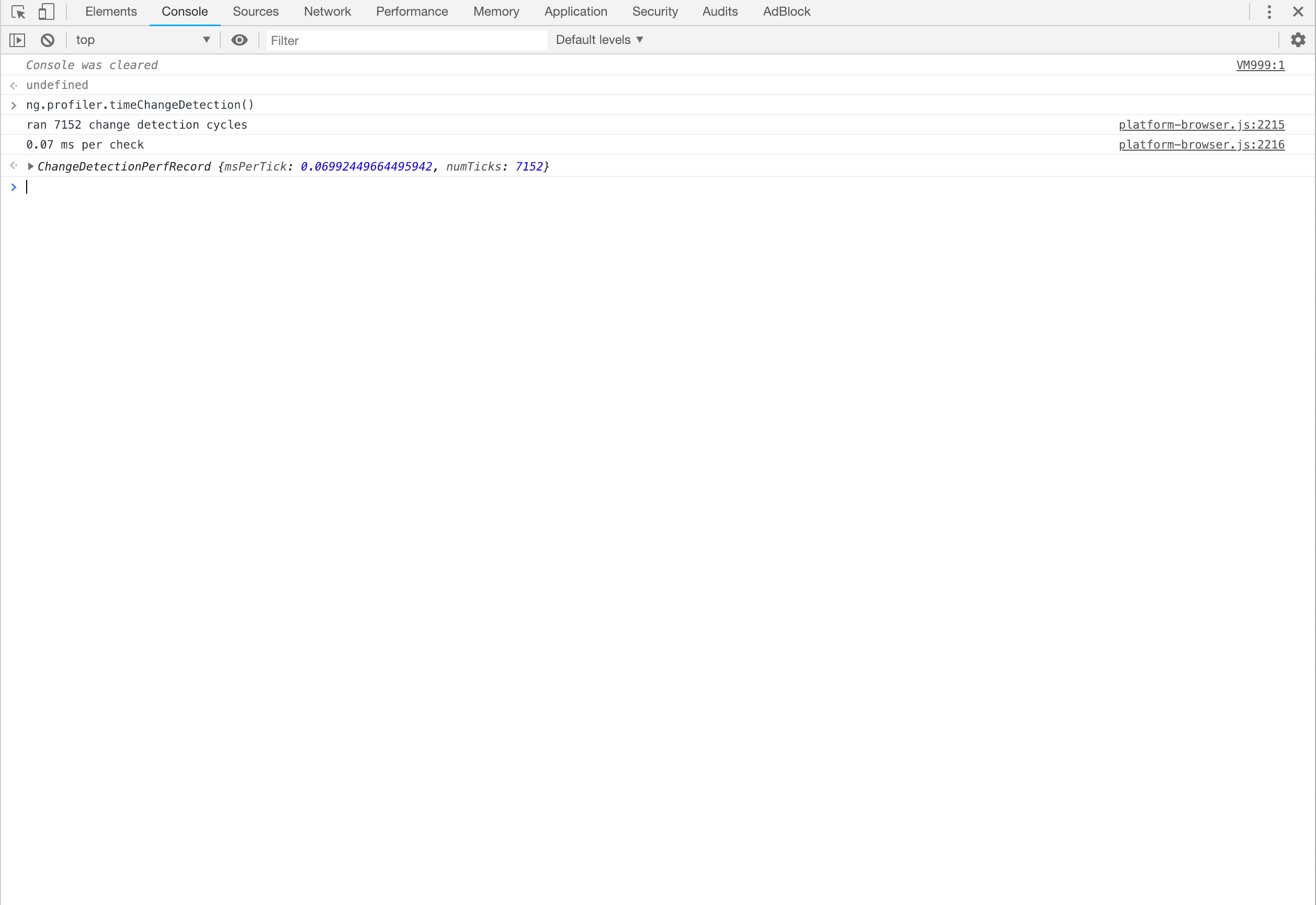A minimalistic web page is depicted, primarily featuring a few small, somewhat illegible coded images. At the top of the page, several black elements act as navigational aids, guiding users to different sections. A standard 'X' button in the upper right corner allows for easy exit. The interface includes various clickable items that help users determine their next steps. The different lines of code, displayed in varying colors like blue, provide additional guidance and functionality. Despite the sparse design, the elements are arranged to assist the user in navigating the site efficiently.